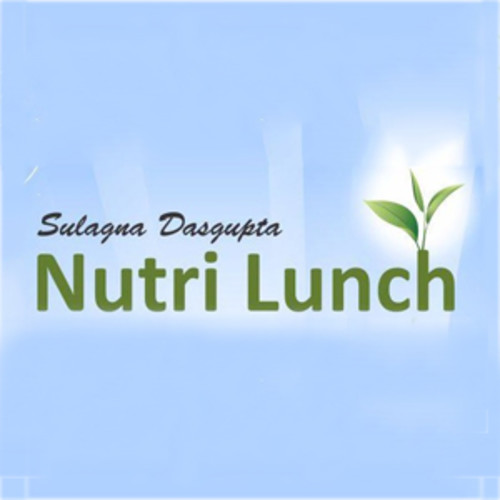The image depicts a likely advertisement with a predominantly sky blue background that transitions into white light at the bottom, giving it a hazy, cloudy effect. Centrally positioned is the name "Salagna Dasgupta" written in black cursive font. Below that, in a larger green font, is the title "Nutralunch" with three leaves sprouting from the top of the "H," which is highlighted by a white blur behind it. The ad appears to promote healthy eating habits and nutritious lunches.